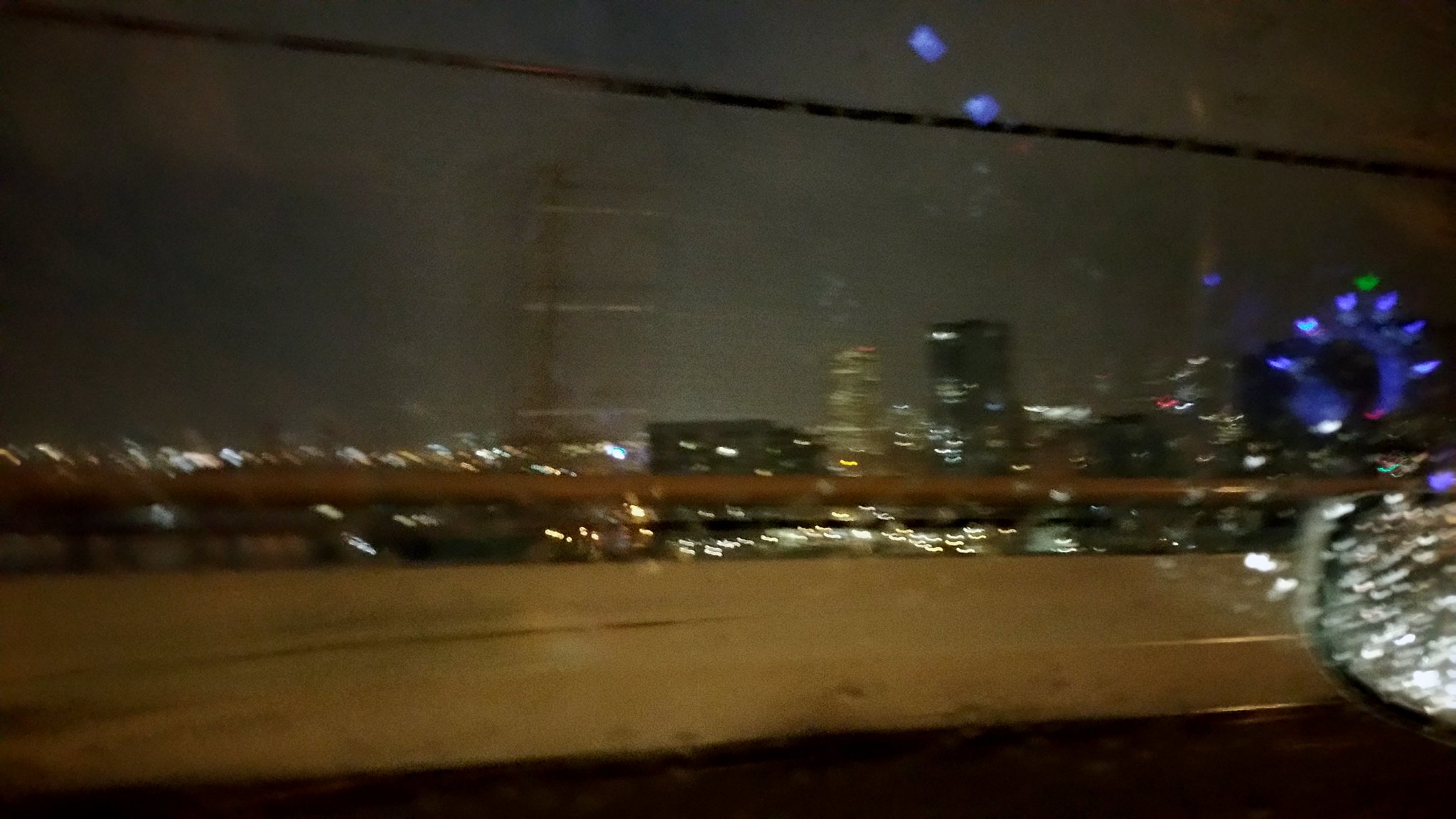Taken at night, this atmospheric photo captures the view through a rain-speckled driver's side window. Reflections of the dimly lit dashboard glow in blue hues on the right side of the image, juxtaposing the gentle outline of the side mirror, also dotted with raindrops, further emphasizing the rainy weather. Beyond the glass, an overpass stretches ahead, overlooking a bustling cityscape. City lights twinkle vibrantly against a backdrop of a dark, cloudy sky, adding a sense of moody serenity to the scene.